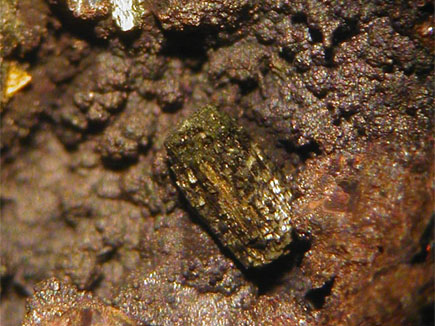This detailed close-up photograph captures an intricate underwater rock formation, likely on a coral reef, showcasing several layers and types of rocks interspersed with mineral inclusions. Central to the image is a notable, oval-shaped, fibrous rock adorned with glistening streaks of gold, possibly fool's gold (pyrite), drawing immediate attention due to its prominent shimmer and textured appearance. The surrounding area consists predominantly of bumpy, craggy rocks, varying in color from reddish-browns to darker hues, suggestive of an igneous origin, likely formed from solidified molten lava. To the right and bottom sections, subtle sparkles hint at additional mineral content. The entire scene is enhanced by the presence of a moray eel peering out cautiously from the coral reef, its greenish-brown head blending seamlessly with the rocky environment, indicating a deeper, shaded underwater setting. The rocks appear slick and wet, implying moisture either from the marine setting or recent contact with water. This vividly detailed snapshot intricately combines geological and marine elements, capturing the elusive beauty of underwater life and mineral richness.